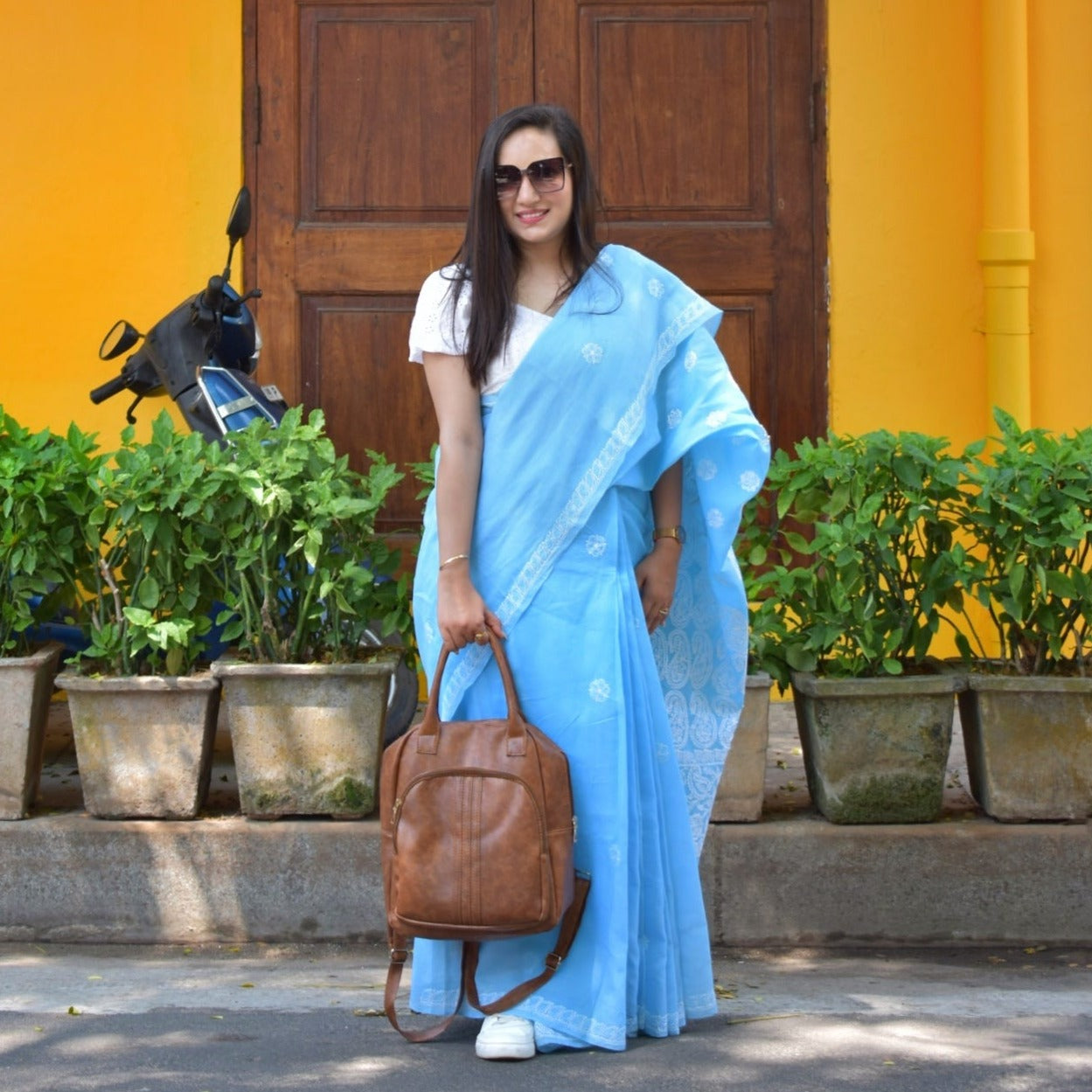The image features a young Indian woman standing outside in dappled sunlight in front of a brightly colored yellow building. She is wearing a traditional light blue sari draped over a white blouse and paired with white sneakers. Her dark brown hair, parted to the side, flows past her shoulders and she is accessorized with oversized designer sunglasses, a gold bracelet, a watch, and additional gold jewelry. In her left hand, she holds a large, light brown leather handbag that doubles as a backpack with visible straps hanging underneath. The backdrop includes a high concrete curb adorned with rectangular stone planters filled with lush green plants. Behind her stands a tall, dark brown wooden double door, flanked by orange walls, and to the left, a blue and black motorized scooter is parked. The photograph captures an essence of elegance and vibrancy, emphasizing the picturesque contrast between the subject's attire and the vividly colored surroundings.